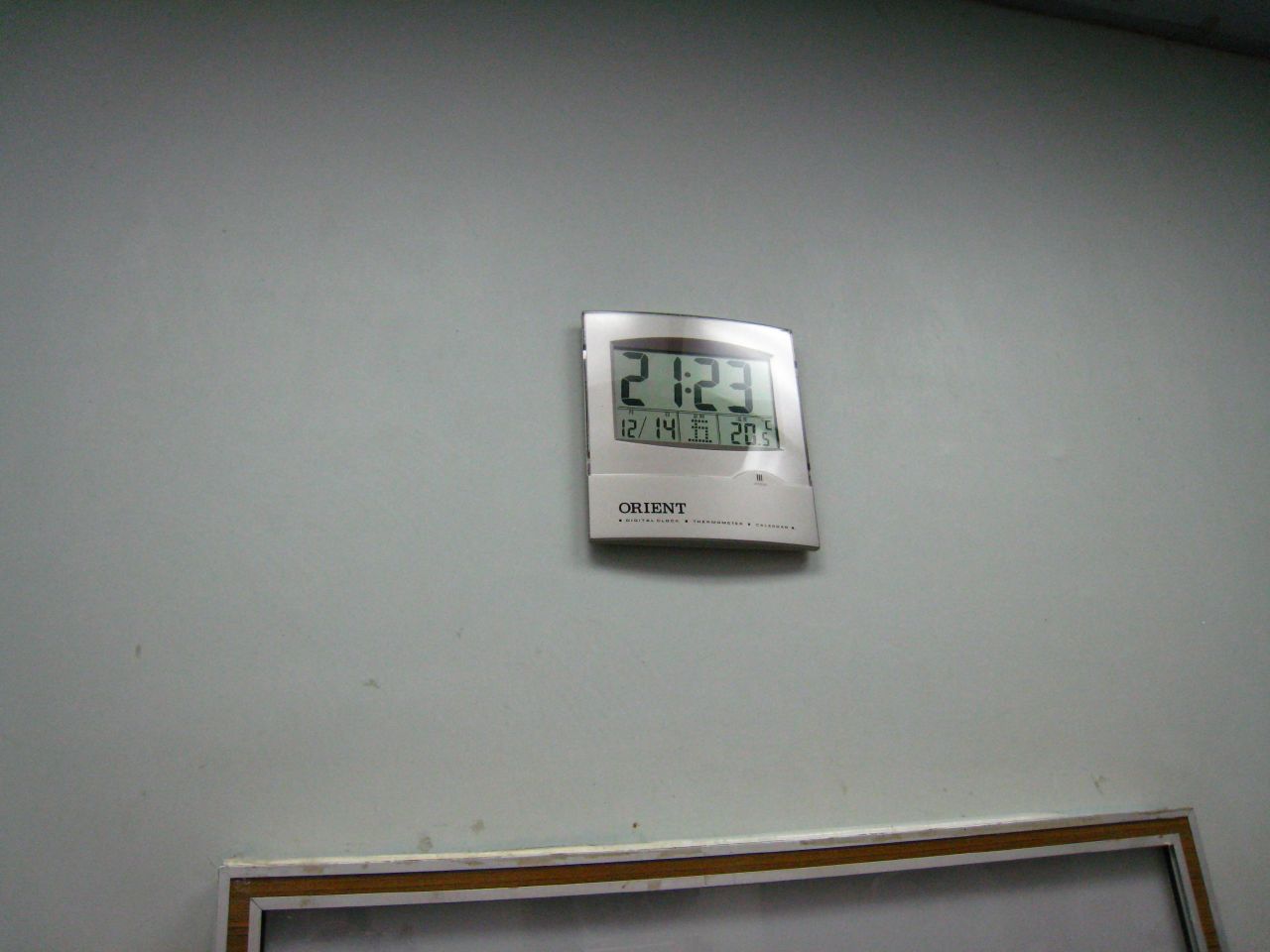In the image, a small, digital clock takes center stage on an otherwise extremely bare and unadorned wall. The wall itself is a greyish hue, contributing to the overall stark and slightly aged appearance of the setting. The clock, which is of the Orient brand, has a greyish-silver casing that blends somewhat with the color of the wall, contributing to its isolated and somewhat incongruous look. The digital display of the clock shows the time as 21:23, with the temperature reading as 20.5°C. Additionally, there is a set of numbers displayed as 12-14, which could potentially indicate the date. The minimalism of the scene draws all attention to the clock, emphasizing its small size and the simplicity of its surroundings.